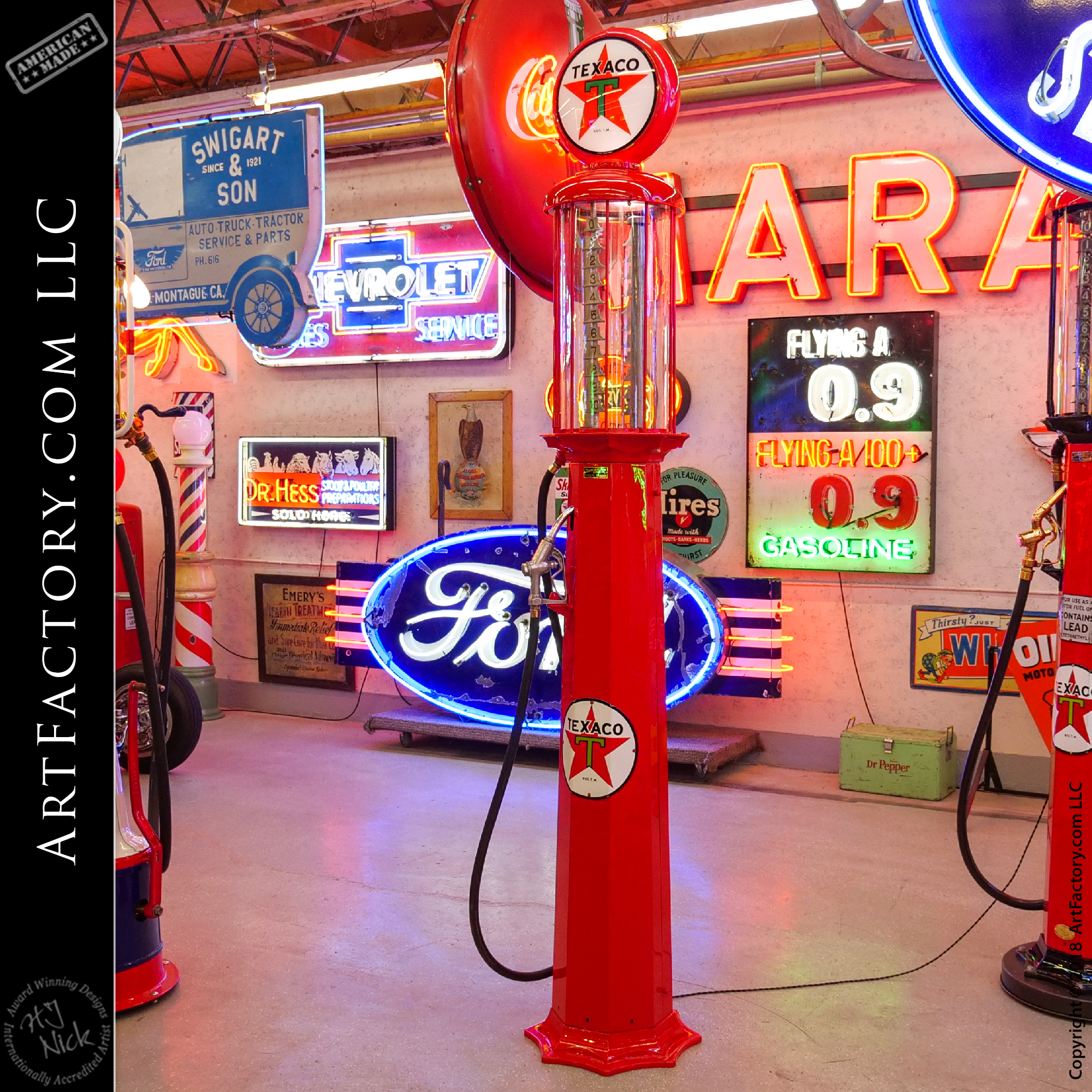The photograph captures an indoor car museum or vintage garage facility, rich with mid-20th century automotive memorabilia. Dominating the center and right of the image are tall, slender Texaco gas pumps from the 1930s, characterized by their bright red color, glass-like tops, and distinctive Texaco logo featuring a white circle with a red star and a 'T'. The pumps are equipped with a black hose attached to their sides. To the left, a vertical black strip displays the text "ArtFactory.com LLC" and "American Made," along with other text in a circular format including "Nick". The background is adorned with an array of illuminated neon signs, including a prominent blue elliptical Ford sign at the bottom, with others advertising Chevron, Chevrolet Service, Swinger and Son Auto Truck Tractor Service and Parts, and Dr. Hess. Additionally, a classic barber pole with red, white, and blue stripes, marked "Flying A 100.90 Gasoline," adds to the nostalgic ambiance. The photograph, with its concrete flooring and square format, offers a detailed and vibrant portrayal of vintage automotive culture.